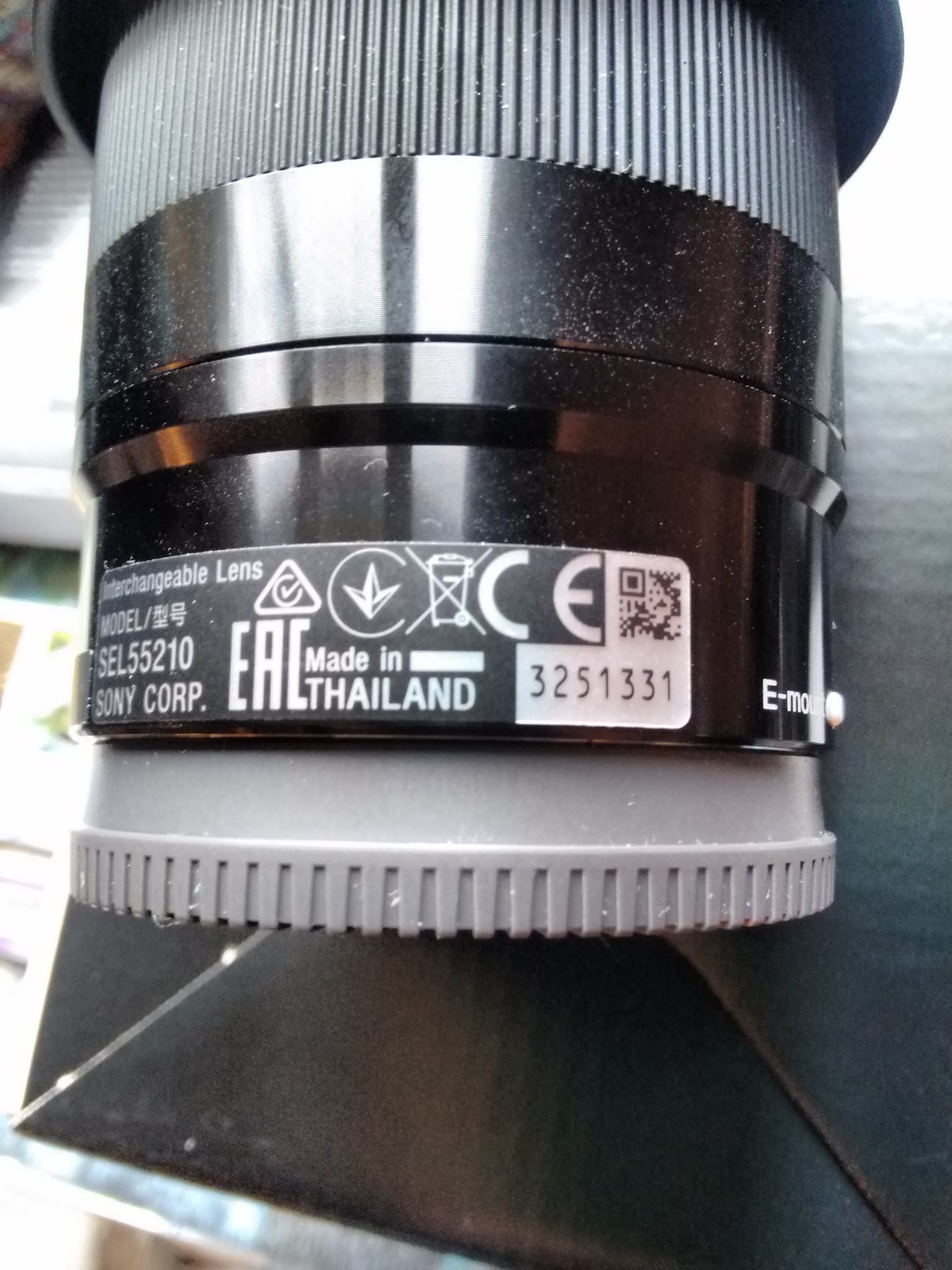The photograph is a close-up, portrait-oriented color image of a Sony interchangeable camera lens, showcasing intricate details of its structure and labeling. The cylindrical object, identified as a lens, features a black horizontal band of plastic encircling its midsection, and a ribbed plastic section at the bottom. The top part of the lens has wider, darker gray vertical ribbing, culminating in a wider black ring that extends out of the frame. A label prominently displayed on the lens reads in white text: "Interchangeable Lens Model//" followed by two Japanese characters. Below, it specifies the model number: "SEL55210," and the manufacturer as "Sony Corp." The label also includes a "Made in Thailand" note, a QR code, recycling symbols, and a crossed-out garbage bin symbol indicating proper disposal instructions. Additional details visible are the regulatory marks "CE" and "EAC". The background includes a glimpse of a black envelope, suggesting the lens is placed on a cluttered desk with other papers and books. This richly detailed image appears to be taken to capture the model information, potentially for purposes of seeking a replacement.